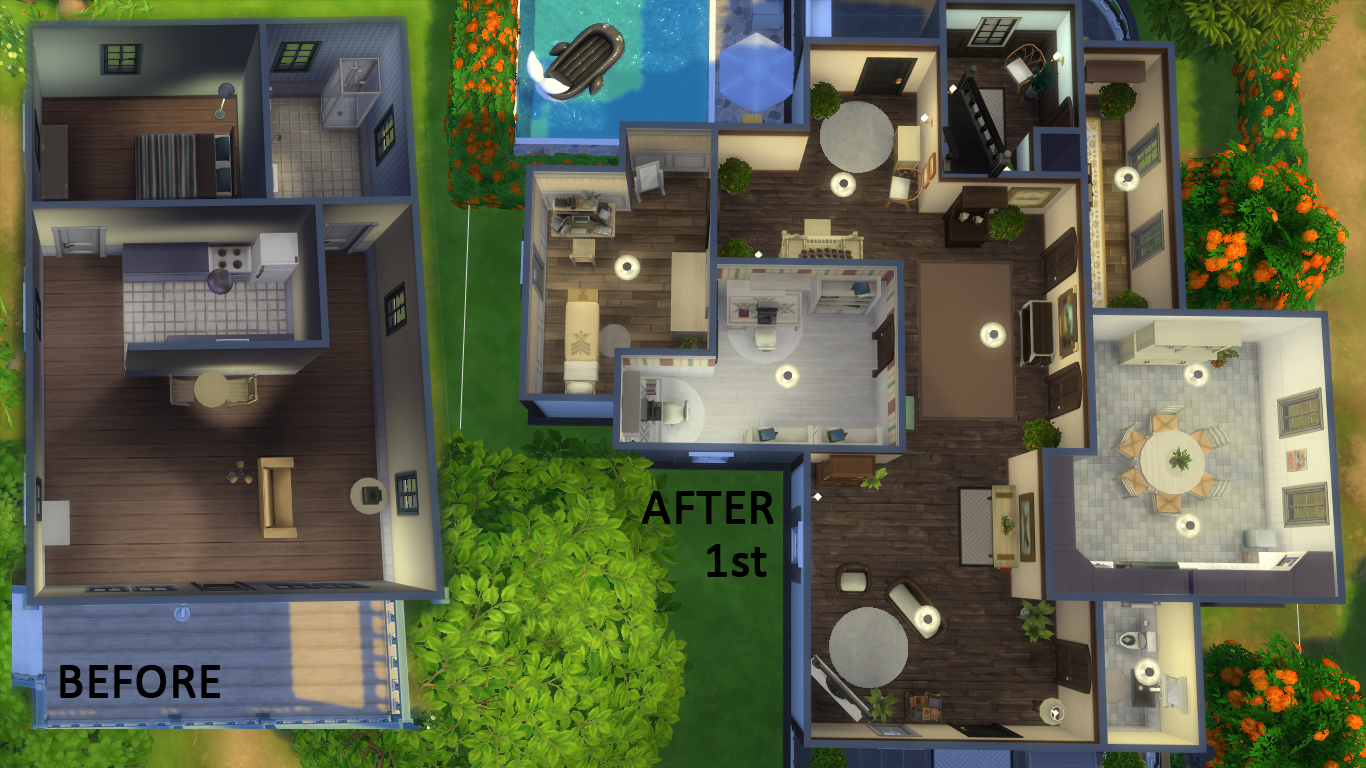The image is a computer-generated top-down view of a floor plan, depicting two different house layouts with their roofs removed for a clear view inside. On the left, marked "before," is a smaller, three-bedroom house. This structure includes a bedroom in the upper left corner, a bathroom in the upper right, a centrally located kitchen with an open floor plan, and a living room situated underneath the kitchen. This house also features a deck at the front.

On the right side of the image, labeled "after first," is a much larger and more complex house with five rooms. It includes an office with two computer desks, various wall hangings, and a lamp, situated in one of the left-side rooms. Next to it is a small bedroom with a cluttered desk. There is also a staircase, a hallway with wood floors and a brown rug, and a living area with a table, chairs, and a couch. The dining room features a table with chairs, a centerpiece, and a cabinet. This house boasts a landscaped yard with green bushes and orange flowers, and a swimming pool located at the back, complete with a black whale floatie and a shade cover. The enhanced design includes more detailed interior furnishings such as a fridge, stove, couch, and additional tables and chairs.